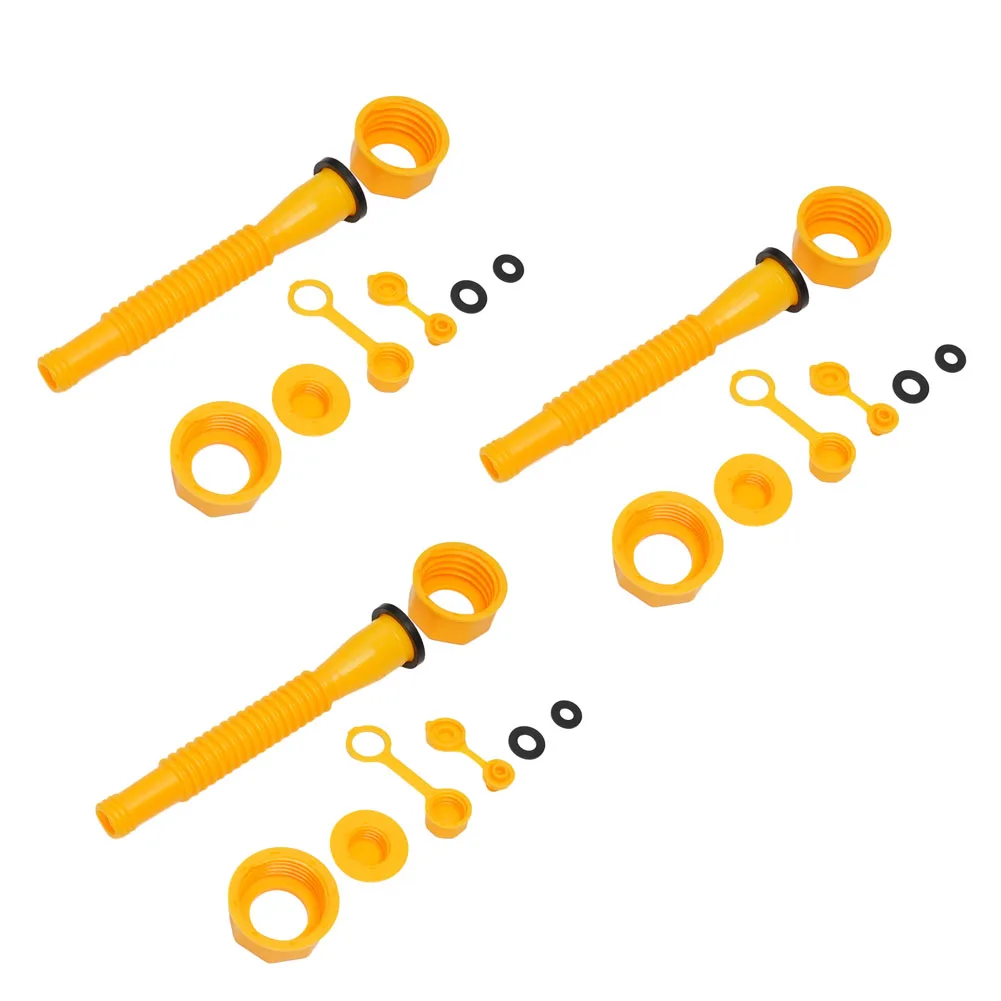The image showcases a detailed product layout of yellow expandable plastic spouts, each accompanied by various fittings and seals, set against a white background. The primary components are three identical sets, each consisting of eight items. Each set features a long yellow plastic tube with expandable segments, reminiscent of spouts used on five-gallon gas cans. At one end of each tube, there is a black rubber gasket and a screw cap designed to secure onto a container. Alongside the spouts, each set includes two black rubber washers, four additional yellow plastic fittings of varying sizes, and multiple cap sizes, all arranged in an orderly fashion. The three sets are laid out to form a triangular shape within the image. The predominant colors are yellow and black, and the repeating pattern suggests this image could be from a catalog or an advertisement.